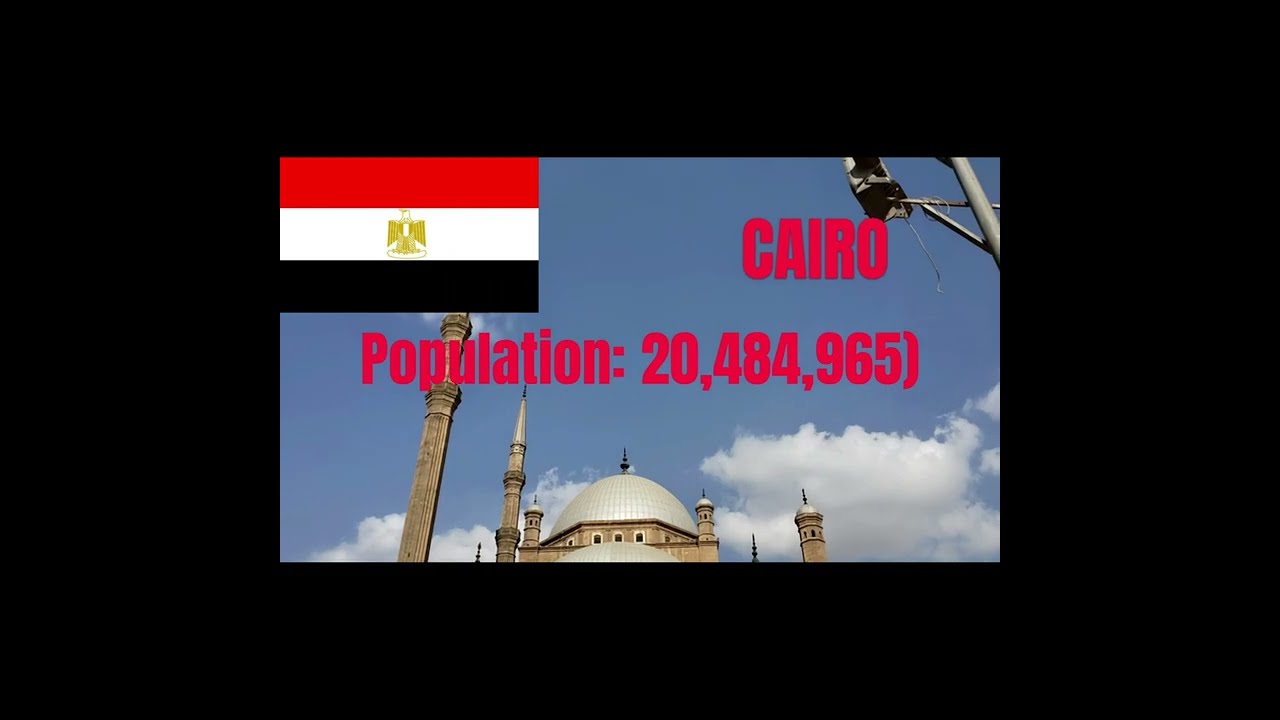The image depicts a color photograph of a Middle Eastern skyline, dominated by a domed building with spires, set against a blue sky scattered with white clouds. The photograph is of horizontal orientation and is inset within a very thick black border, making the central image appear smaller. In the upper left-hand corner, there is a prominent depiction of the Egyptian flag, featuring horizontal stripes in red, white, and black, with a golden eagle in the center of the white stripe. On the right side of the image, a streetlight (or possibly a security camera) is visible, contributing to the urban ambiance. Bold red text at the top declares "CAIRO," with the population figure "20,484,965" in smaller red uppercase print directly below. The overall composition emphasizes the architectural and cultural elements of Cairo, encapsulated within a striking, bordered frame.